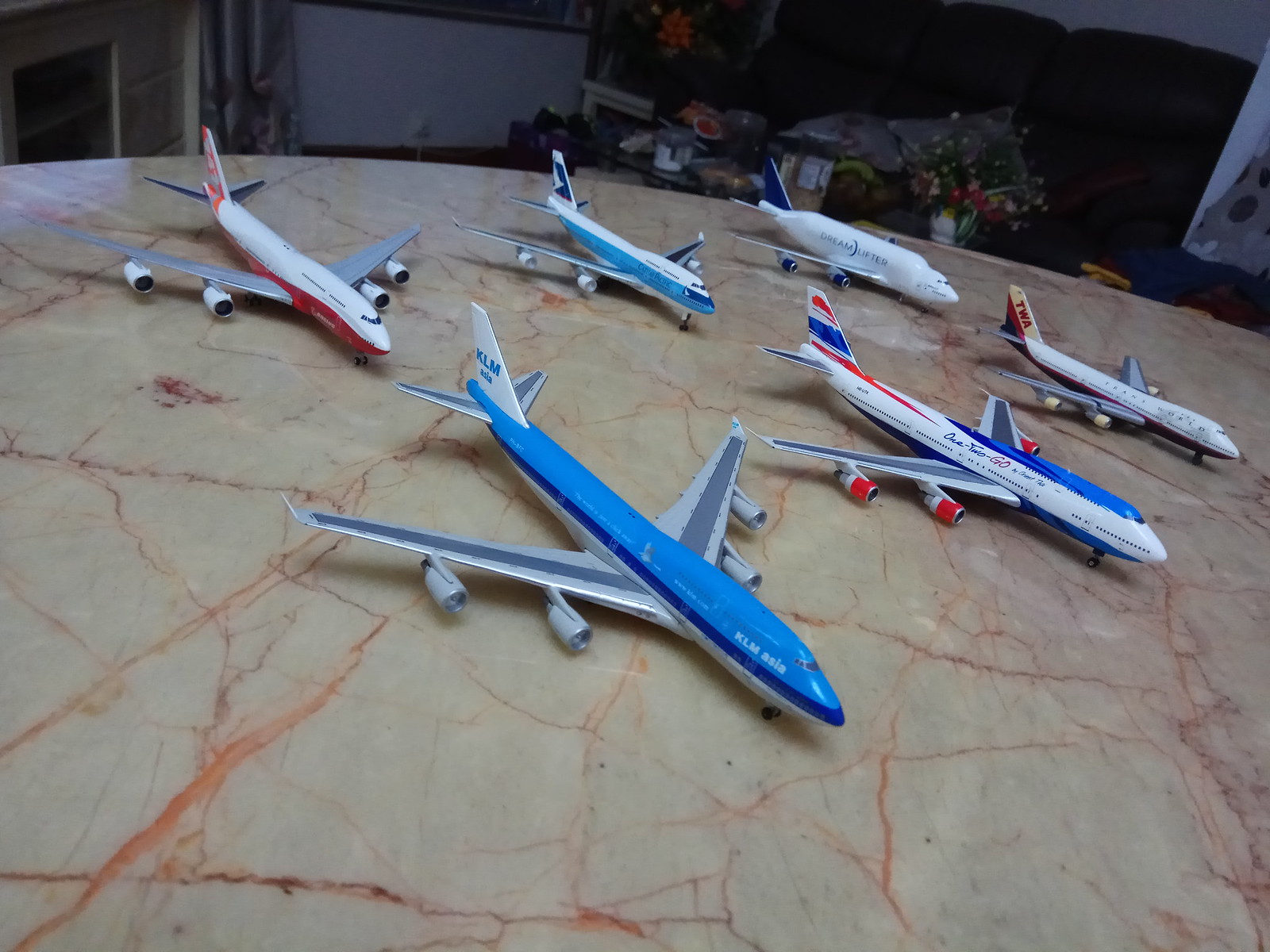The image depicts a collection of six distinct model airplanes displayed on a large, round beige marble table. The marble table, adorned with amber-colored veins, dominates the lower two-thirds of the image and spans from the left to the right edge. Each model plane is uniquely designed and positioned with their noses pointing towards the bottom right of the frame, and their tails angled towards the top left.

In the foreground on the left, a bright blue model airplane with dark blue stripes and white tails is prominently labeled "KLM Asia." Adjacent to it sits a model bearing a white and red color scheme with a grey and red striped tail pattern, featuring two silver wings and four white engines.

Next, moving rightward, is a blue, red, and white airplane, adorned with lettering that is partially legible, hinting at the word "go." Further back, an all-white airplane has blue, illegible writing and a dark blue tail. 

To the right, another model plane draws attention with its light blue top, white bottom, and a thin dark royal blue stripe in between. This model's wings are silver with darker centers, and it features four jet engines underneath its wings.

Additionally, there's a model with blue, white, and silver coloring; its engines are red and white, and the tail hosts a mix of red, white, and blue patterns. The final plane, set farthest back, is predominantly white on top and burgundy on the bottom, with yellow and silver engines and a tail featuring red lettering on a yellow background. The detailed tabletop scene is set against a background of a white desk, a tiny white wall, a black couch, and a cluttered table visible behind the marble surface.